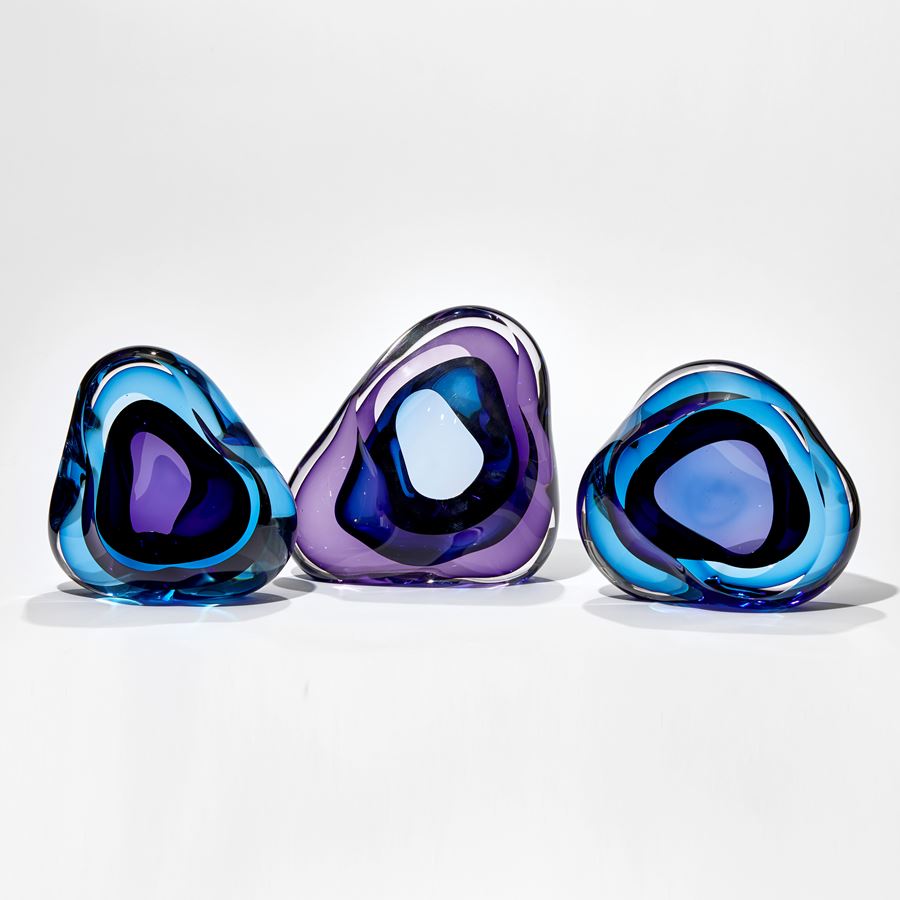This digital art image features three translucent, jelly-like shapes arranged against a white background. The objects have a distorted triangular form with a blend of vivid colors, giving off a glassy, almost crystalline appearance. The leftmost shape has an outer region of blue with a core that shifts from purple to black. The central figure predominantly showcases a purple exterior, transitioning to blue and culminating in a white core. The rightmost object mirrors the left's blue-dominant outer area but houses a core of light purple mingled with black. Shadows beneath these shapes are rendered in light gray, enhancing their three-dimensional, semi-transparent character.